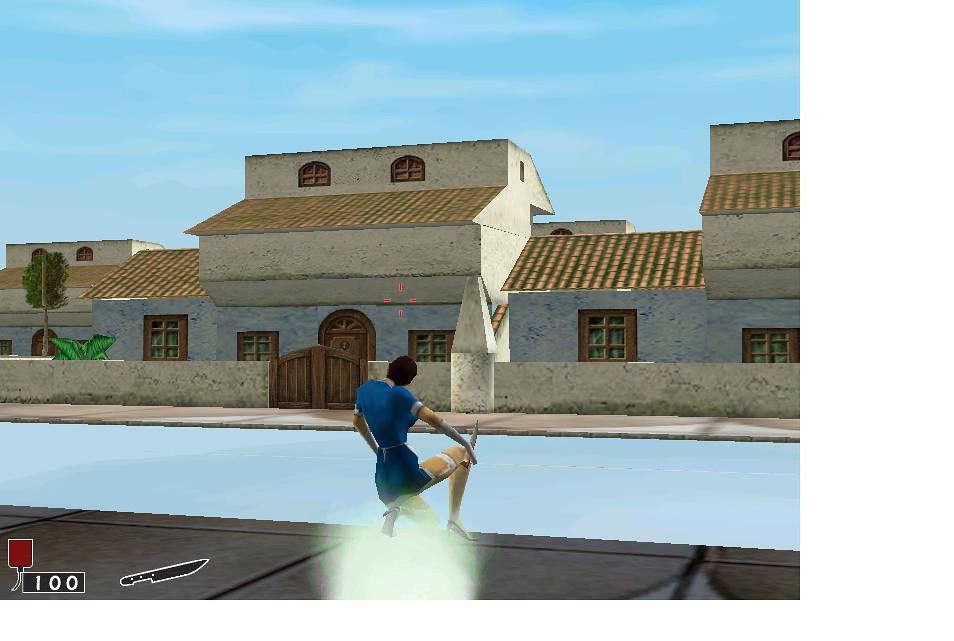The image appears to be a low-polygon, 3D model from a vintage video game, possibly from the PS1 or PS2 era. It features a detailed scene with a blue sky overhead and an older, multi-story beige brick building with a brown roof, wooden-framed windows, and several doors on the lower level. A significant detail is the cement brick wall with a wooden gate in the center that surrounds the building. 

In the foreground, a character, likely female, is depicted kneeling or bending down near what appears to be a street marked by light blue lines, initially mistaken for a body of water or a pool. The character seems to be wearing a blue outfit, possibly a romper, with heels and a garter belt, and holds a knife in her right hand. 

On the bottom left corner of the image, there is a red box next to a brown box displaying the number "100," which is indicative of a health or status bar common in video games. Accompanying this is a diagram of a knife outlined in white. The scene is further illuminated by a light source flashing at the bottom middle of the image.

The background architecture is reminiscent of Mexican or Hispanic-inspired designs, with residential concrete buildings and an essential mix of wooden gates and cement fences. Adding to the overall setting are elements that suggest the game involves violence, as indicated by the red target sign often associated with shooting games, but here knives appear to be the primary weapons.